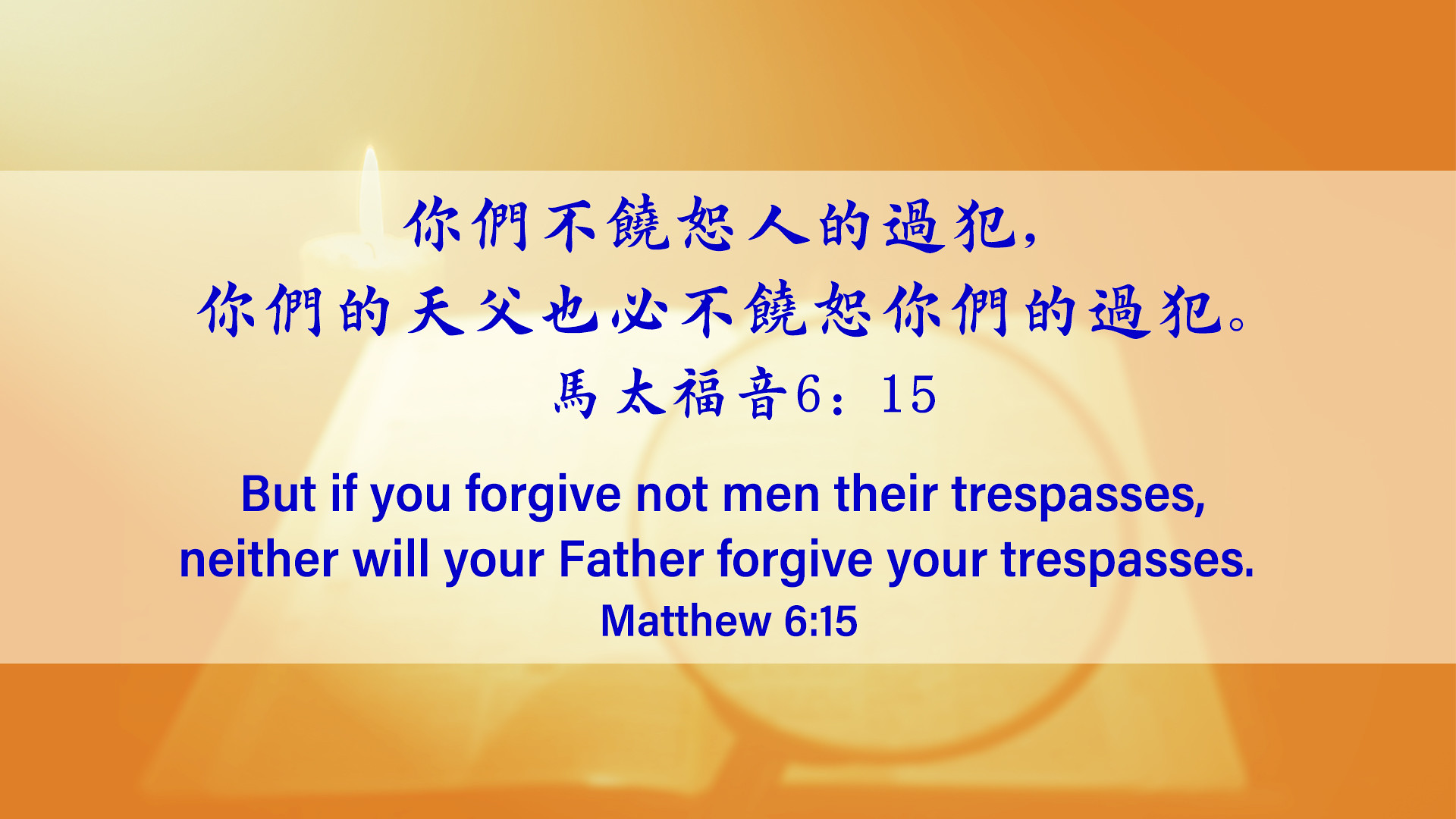This wide rectangular image features a religious quote from the Bible, Matthew 6:15, displayed prominently in both an Asian language and English. The background is a rich gradient transitioning from a pale yellow in the top left corner to a deep orange on the right, creating a warm and inviting atmosphere. A faint image of a magnifying glass shadow hovers over a square-shaped yellow object in the bottom center, while the hint of a candle can be seen at the top left, adding subtle details to the composition. The quote, "But if you forgive not men their trespasses, neither will your Father forgive your trespasses," is highlighted in bright blue text within a long, thick, translucent light yellow rectangle that separates it from the vibrant background, providing clarity and emphasis.